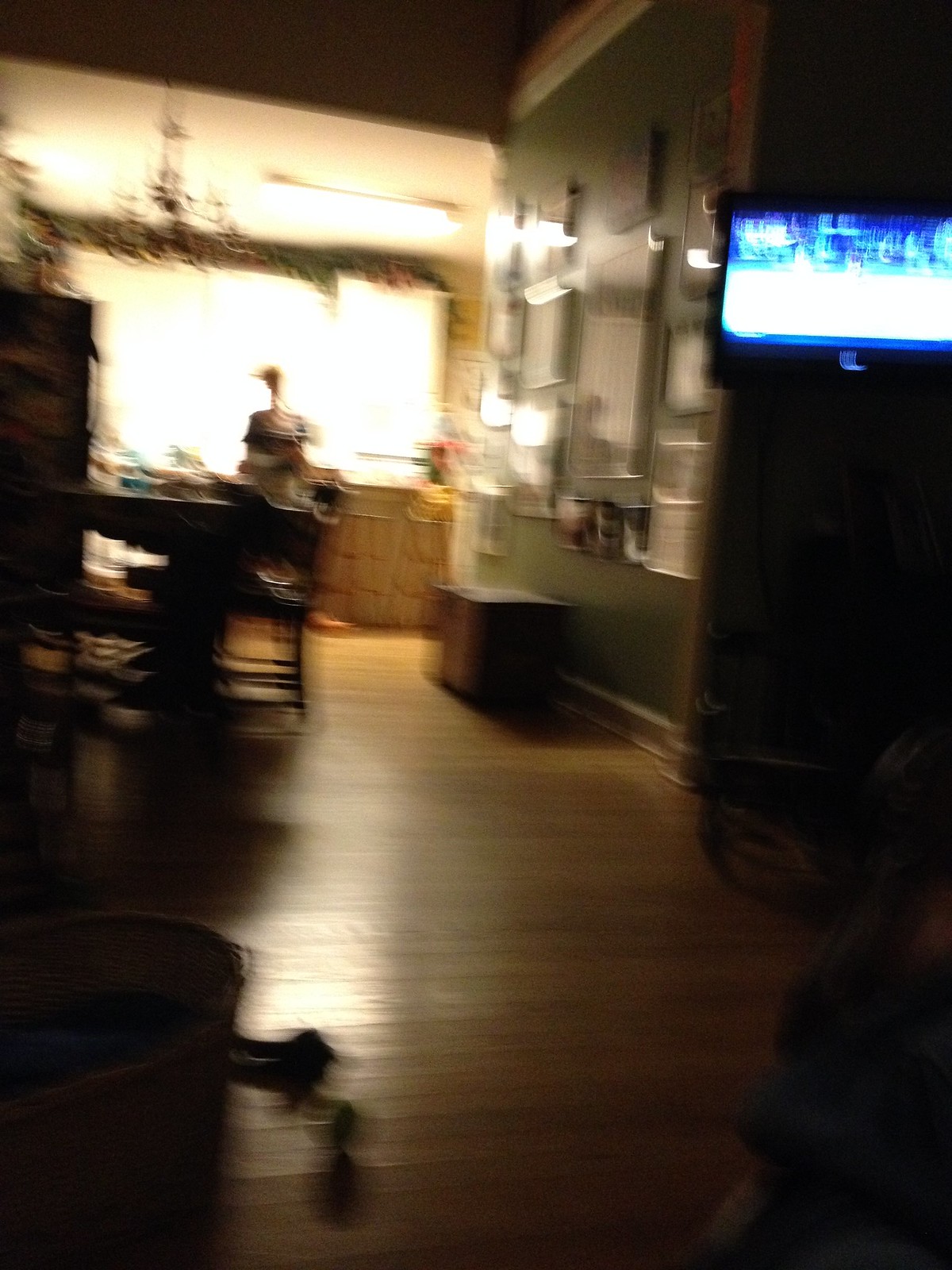The photograph depicts a dimly lit room with a significant amount of light coming from a large window, partially covered with greenery at the top, which creates a stark contrast with the otherwise dark interior. The room seems to be a cafe or restaurant, possibly closing up, with various elements slightly out of focus. A white and blue TV, mounted on the wall to the right, emits a bright light, presumably displaying a sports game. The surrounding area includes a wooden bench and several frames of different sizes on a green wall. On the lower left side, there's a round object that seems to be some sort of woven basket or hamper. 

In the foreground, a desk or table with scattered papers and an array of items rests under the window. A chest can be seen against the white wall on the right, along with a series of indistinguishable pictures hanging above it. The wooden floor extends to bar stools aligned along a wall. Near the cashier counter, a person is faintly visible. There is also an overhead chandelier that adds to the room's lighting, and a drink machine or fridge is noticeable to the left. The overall scene is blurry and out of focus, making some details hard to discern, but the ambiance of the room indicates a cozy and bustling yet somewhat disorganized space.